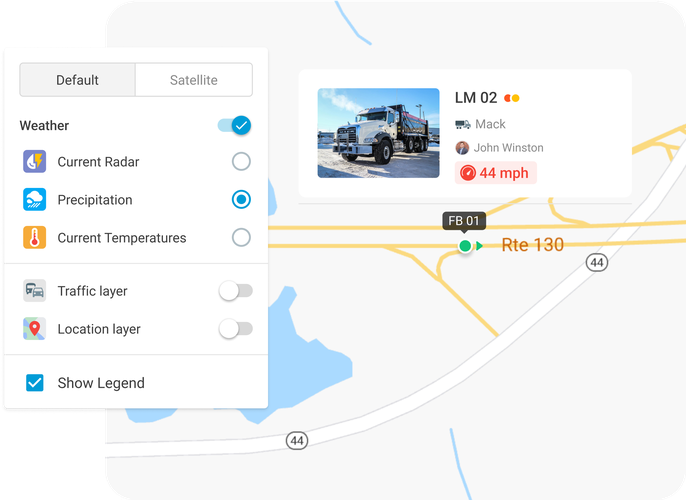This image is a detailed screenshot of a website displaying a sophisticated tracking system. In the background, a road map—provided by Google Maps or a similar service—serves as the primary display. Superimposed on this map is a small white rectangle pinpointing a specific location where a user is currently active. 

A large dump truck with a white cab prominently labeled "LM02" sits at the pinpointed location. The truck is identified as a Mack model, and its driver is John Winston, who is driving at a speed of 44 miles per hour. 

On the left-hand side of the image is a larger white rectangle housing various clickable options for different display settings. At the top, there is a tab selected for "default," which shows the standard map view. Alternatively, users can choose to view a satellite image of the area. Below this, several other toggles are visible: 

- "Weather," which is currently turned on.
- "Current radar," which is not toggled.
- "Precipitation," which is toggled on.
- "Current temperatures," which is not toggled.
- "Traffic layer," which is off.
- "Location layer," which is also off.

There is also a checkbox labeled "show legend" at the bottom of this section, which is currently checked.